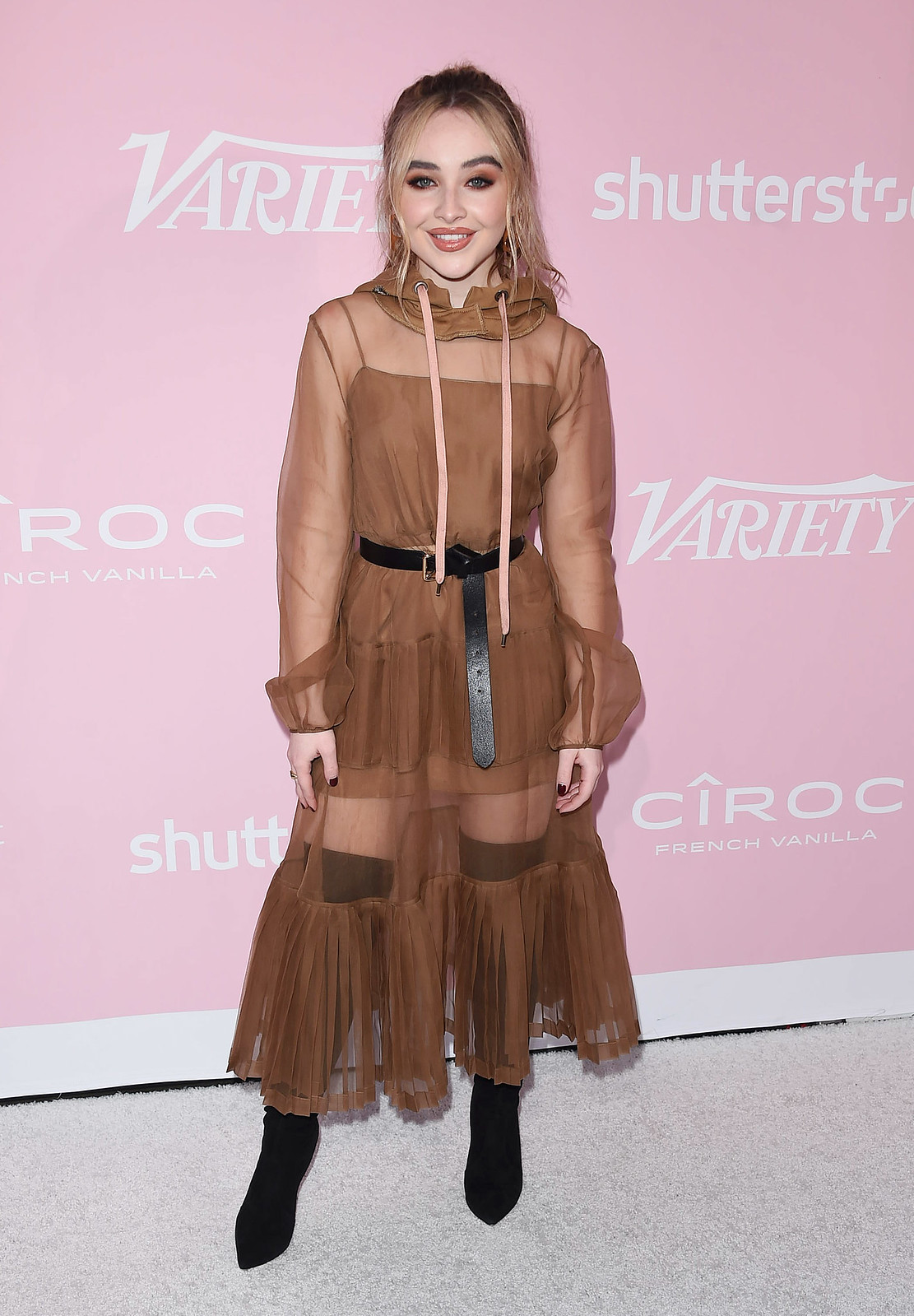The image features a young female entertainer posing before an event, standing in front of a pink backdrop with various logos, including Variety, Shutterstock, Ciroc, and French Vanilla. She is wearing a brown, hooded dress with gauzy, see-through sections on the arms, upper chest, and legs. The body of the dress is a darker brown with thin stripes beneath the sheer portions. Her ensemble includes a black belt cinching her waist and a pair of high black boots that reach past her knees. She accessorizes with large gold earrings, and her makeup features a brown to peach color theme with matching lipstick and eyeshadow, accentuated by black eyeliner. Her hair is a medium brown with lighter highlights, and she stands confidently on a light gray floor, with a hint of a smile showcasing the top row of her teeth. Her arms are down by her sides, feet slightly apart, and her overall look is completed with prominent cheekbones and black-painted nails.